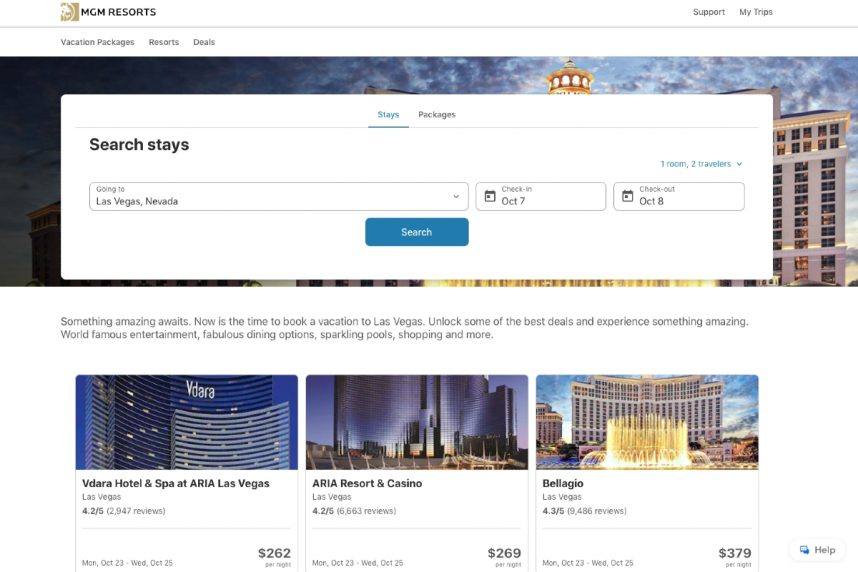This is a vibrant color screenshot of the MGM Resorts webpage, prominently featuring the MGM Resorts logo with a gold and white lion at the top. The layout includes various navigation options such as "Vacation Packages," "Resorts," "Deals," and "Support," along with user-specific selections like "My Trips." The search tool is prefilled with a trip to Las Vegas, Nevada, with check-in on October 7 and check-out on October 8, for one room accommodating two travelers. 

The page highlights the call to action: "Something amazing awaits. Now is the time to book a vacation to Las Vegas," encouraging potential visitors to "unlock some of the best deals and experience something amazing," with mentions of "world-famous entertainment, fabulous dining options, sparkling pools, shopping, and more."

A prominent photograph of the Vdara Hotel and Spa at Aria Las Vegas showcases the luxury accommodations. Vdara is noted for its 4.2 average rating out of 5, based on 2,947 reviews, with room rates from Monday, October 23rd through Wednesday, October 25th at $262 per night.

Additionally, the Aria Resort and Casino, Las Vegas, is highlighted with an average rating of 4.2 out of 5 from 6,663 reviews, offering room rates for the same dates at $269 per night. The Bellagio, Las Vegas, another prominent feature, boasts an average rating of 4.3 out of 5 from 9,486 reviews, with room rates of $379 per night for the corresponding dates.